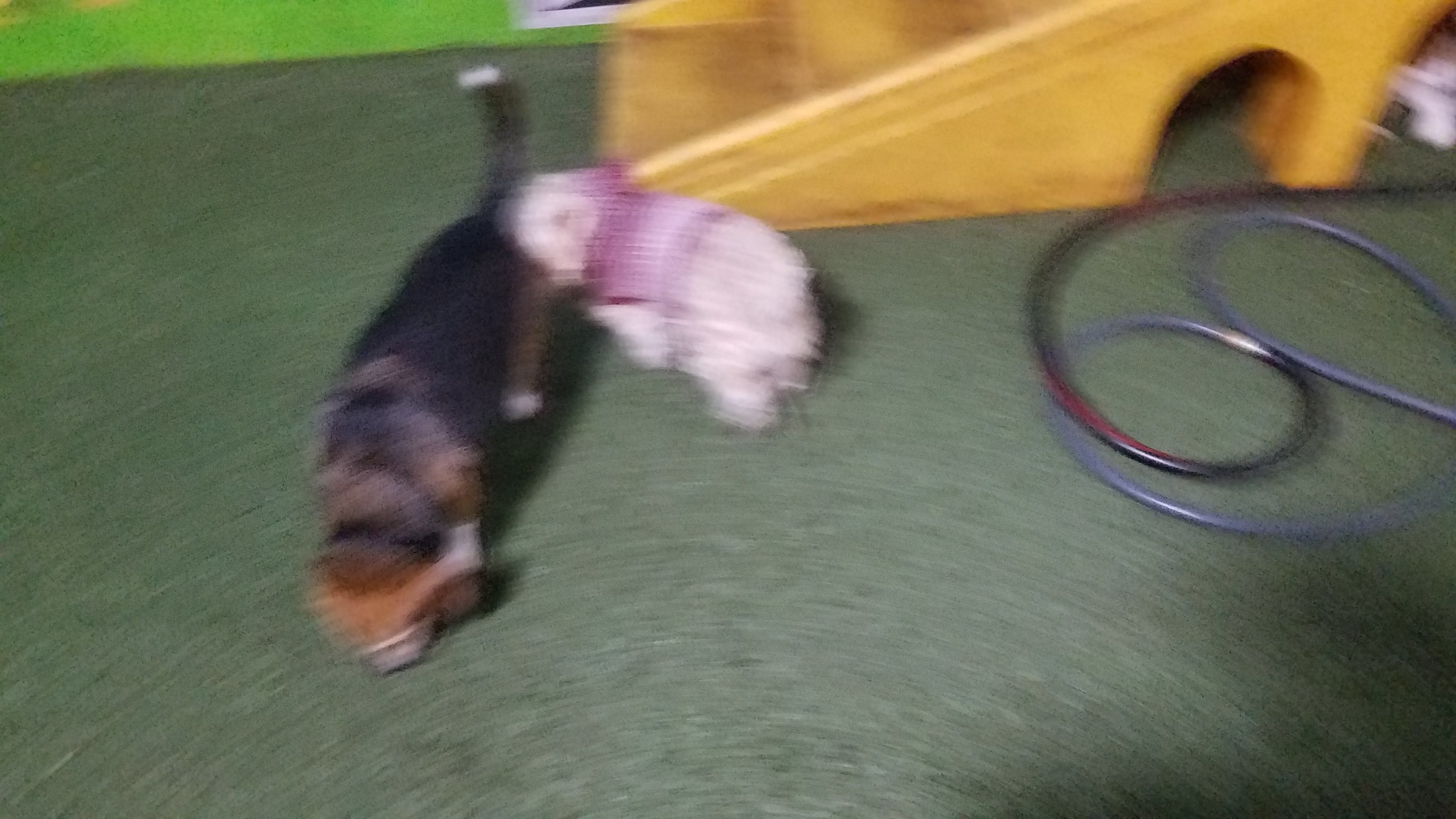The blurry image captures a lively scene in a dog playpen area characterized by its dark green carpet and lime green walls. At the center, two dogs engage in typical canine behavior. On the left, a slightly larger dog resembling a beagle, with tri-colored fur including a black back and a white-tipped, black tail, has its head to the ground as if sniffing something. Its floppy ears and coloring are distinctive, even in the blurred image. A smaller white dog with fluffy fur, possibly a Maltese or a West Highland Terrier, appears to be sniffing the first dog's butt. This smaller dog is adorned with a pink-to-white gradient jacket. In the background, a wooden staircase with a small tunnel beneath it acts as an activity structure for the dogs. Additional details include a coiled cable situated near the staircase and various dog toys scattered around, indicating a playful environment for the pets. The overall image, while unfocused, conveys a sense of dynamic interaction and a comfortably equipped play area for dogs.